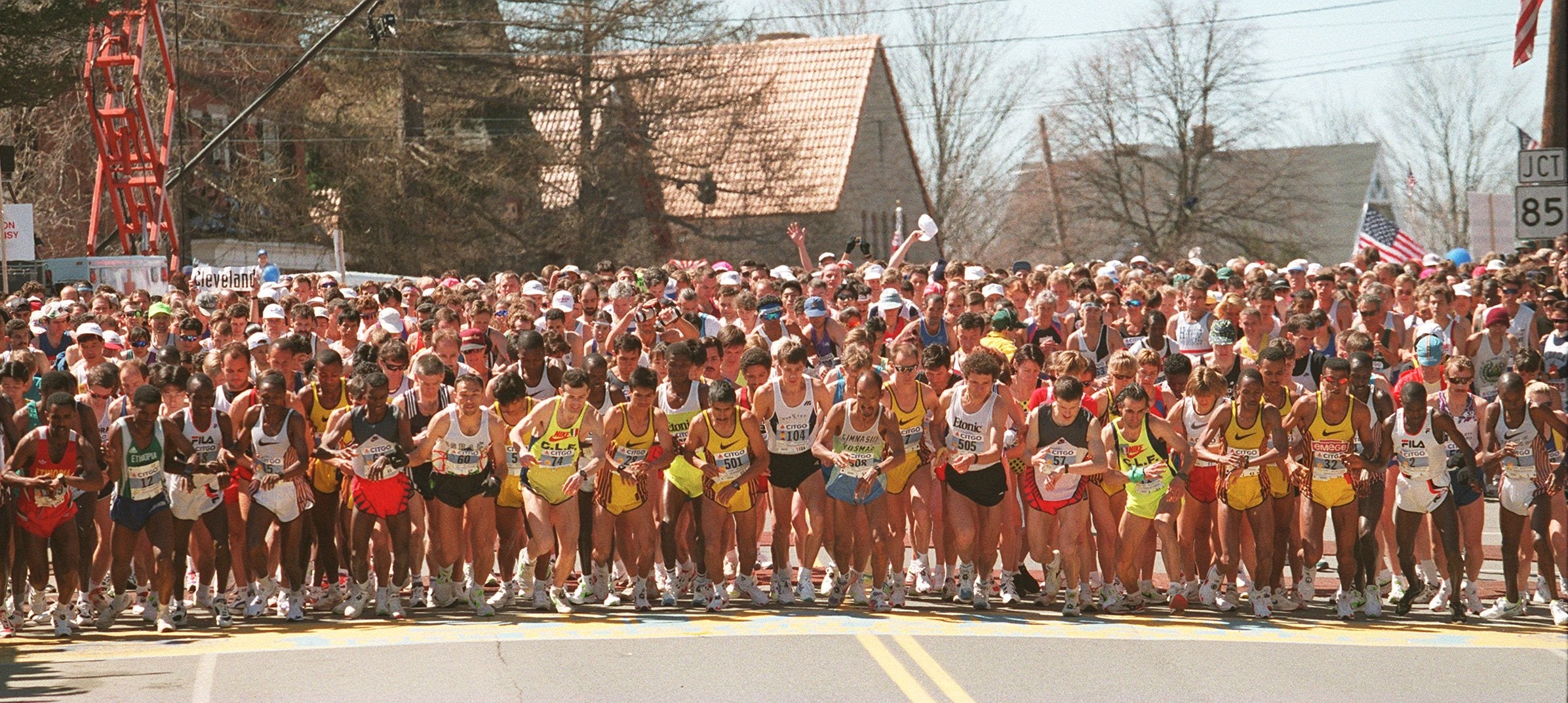The photograph captures the energetic start of a large marathon, with hundreds of runners at the beginning of the race, just taking their first steps after the starting pistol. The image, displayed in landscape mode, showcases a diverse crowd of athletes of varying skin tones dressed in colorful running gear, including shorts, tank tops, and athletic shoes. At the forefront, we see the yellow road lines on the black asphalt, indicating they are on a street or highway. The runners, focused and ready, have their legs in motion and arms flexed as they face the camera. 

In the background, the scene is set on a sunny fall day, evidenced by the leafless trees. There are several peaked-roof houses, electrical wires crossing the image horizontally, and a prominently displayed street sign that reads "Junction 85." An American flag partially visible suggests a patriotic element to the event. Additionally, a mysterious red structure, possibly for camera equipment, can also be seen, adding to the race day atmosphere. The overall mood is bright and filled with anticipation.